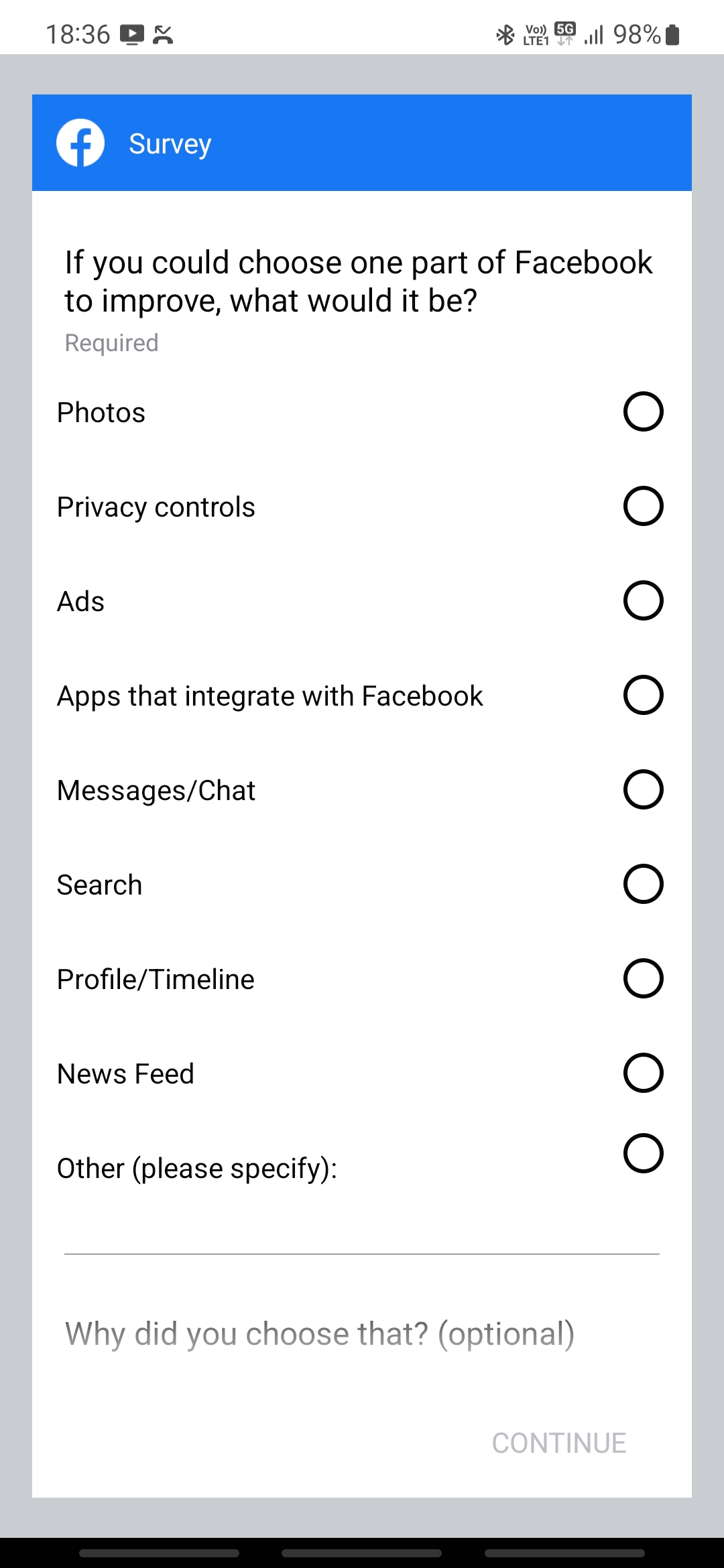The screenshot likely from an iPhone displays a survey interface for Facebook with various features listed for user input. The device's status bar at the top shows the time as 18:36, battery life at 98% charged, and other standard icons. Below it, the background features a thin gray line with a light to medium blue strip at the very top, where the Facebook "F" icon is visible alongside the word "survey" in white text.

The main content area, set against a white background, presents the question: "If you could choose one part of Facebook to improve, what would it be?" This question is marked as "required" in gray lettering below. There is a list of options with corresponding radio buttons to the right of each item. The options include:

- Photos
- Privacy controls
- Ads
- Apps that integrate with Facebook
- Messages/Chat
- Search
- Profile/Timeline
- News feed
- Other (please specify)

Underneath this list, a prompt appears: "Why did you choose that?" with "(optional)" noted in parentheses. Finally, a "Continue" button is situated at the bottom of the screen.